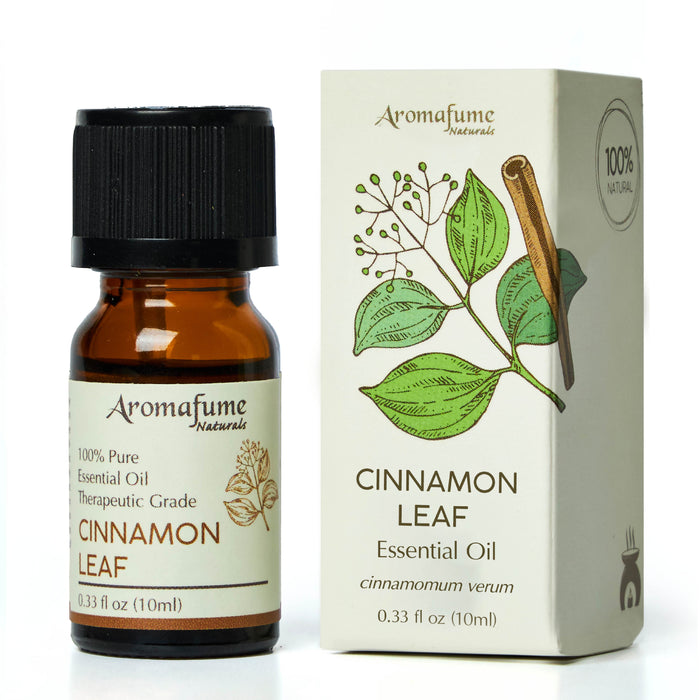This image displays an essential oil product named AromaFume Naturale Cinnamon Leaf. On the left side, there's a small amber-colored glass bottle with a black top. The bottle features a beige label with bronze-colored text stating "Aroma Fume Naturale, 100% Pure Essential Oil, Therapeutic Grade, Cinnamon Leaf, 0.33 fluid ounces, 10 milliliters." The label also includes an illustration of a cinnamon leaf. To the right, there's a light beige box, branded with the title "Aroma Fume Naturale," accompanied by a visually appealing picture of green leaves alongside a cinnamon stick. The box also specifies "Cinnamon Leaf Essential Oil, 0.33 fluid ounces, 10 milliliters," and carries a "100% Natural" stamp on the side. This detailed presentation highlights the product's natural and therapeutic qualities, making it visually enticing for potential buyers interested in aromatherapy essentials.